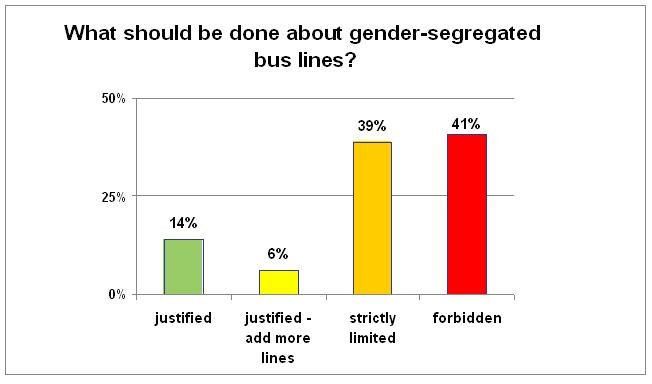The image displays a PowerPoint-style slide featuring a bar graph against a white background with black text. The title at the top reads "What should be done about gender segregated bus lines?". The vertical axis on the left is labeled with percentages, marked at 0%, 25%, and 50%. The horizontal axis along the bottom lists four options: "Justified," "Justified - Add More Lines," "Strictly Limited," and "Forbidden." Each option corresponds to a colored bar: green for "Justified" with 14%, yellow for "Justified - Add More Lines" with 6%, orange for "Strictly Limited" with 39%, and red for "Forbidden" with 41%.